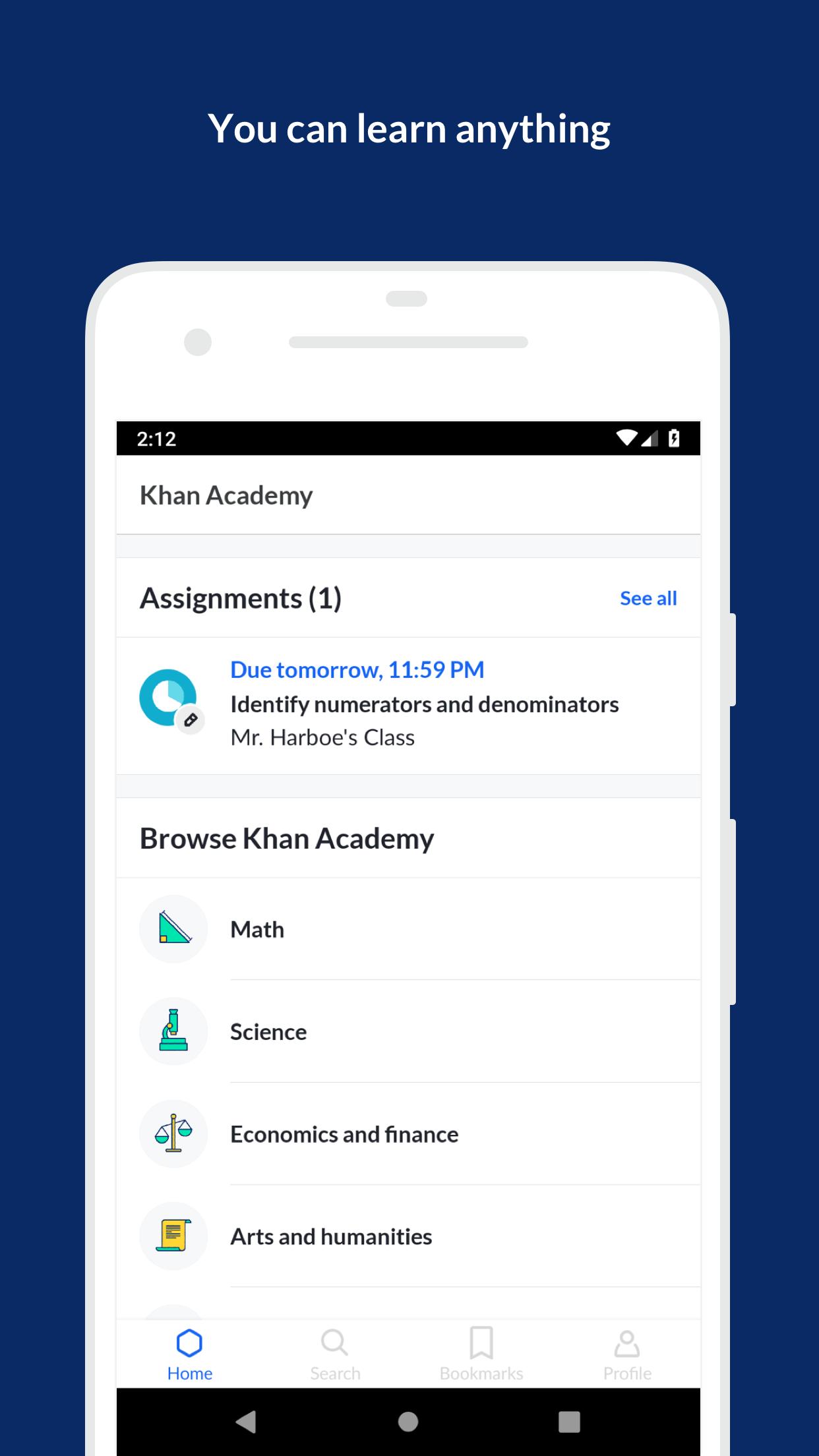**Caption:**

This image captures an informational slide from a website showcasing a product offering from Khan Academy. The background is primarily blue at the top, featuring the motivational phrase "You can learn anything" in small white letters, centered prominently. The focal point of the slide is a white iPhone displaying the Khan Academy app.

On the screen of the iPhone, the app's interface is visible. The header reads "Khan Academy" with "Assignments 1" positioned in the top-left corner, and on the right, there is a "See All" link in small blue letters. Below this header, the section titled "Due Tomorrow, 11:59 p.m." highlights an assignment titled "Identify numerators and denominators." This is followed by the label indicating the teacher's class.

Further down the screen, several navigation options are listed, including "Browse Khan Academy," "Math," "Science," "Economics and Finance," "Art," and "Humanities." At the bottom-left corner, a blue "Home" button is visible. The very bottom of the screenshot reveals the iPhone's physical navigation buttons, including a left-pointing arrow and a central "Home" button.